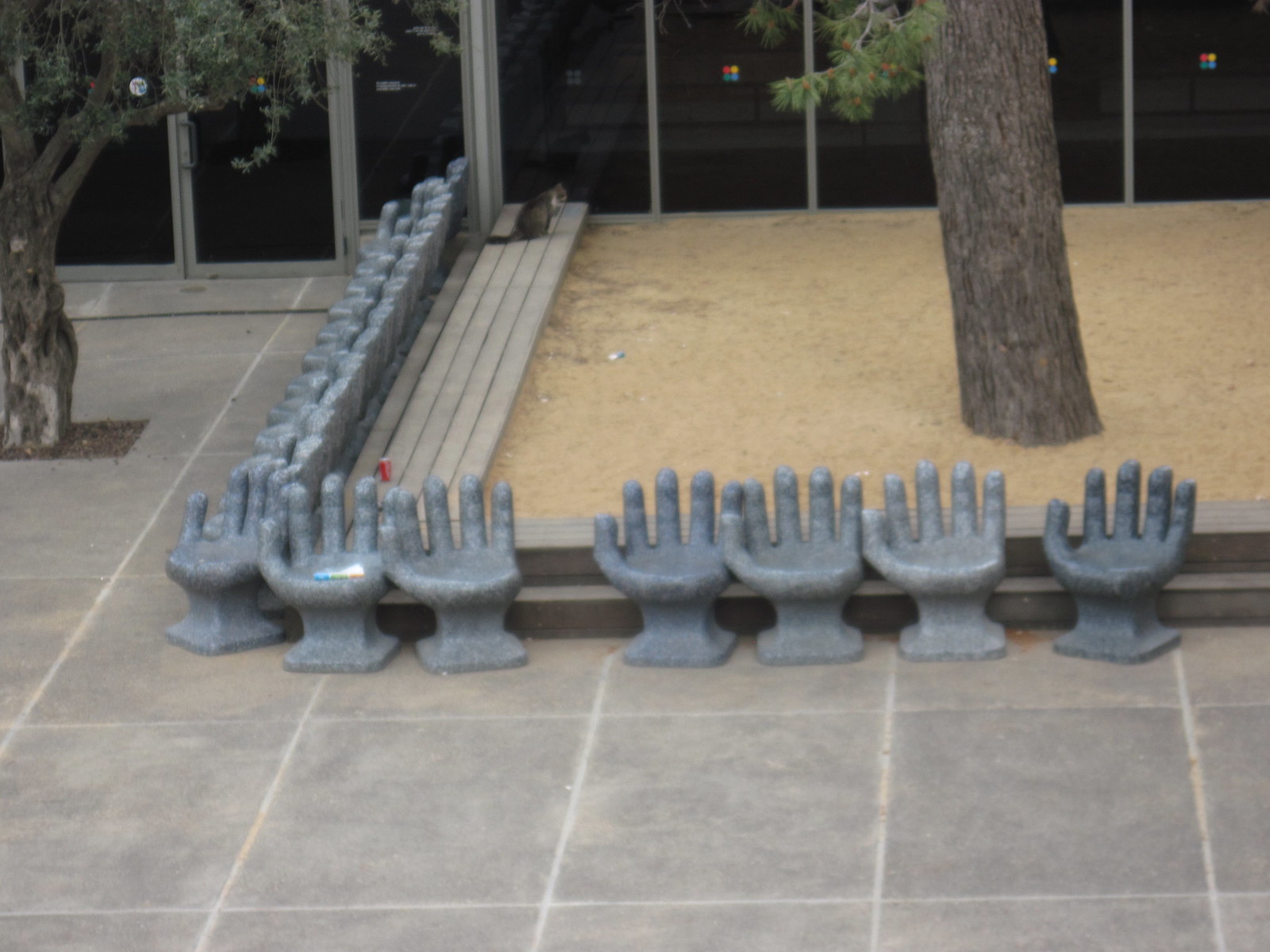This photograph captures an outdoor seating area adjacent to a building with floor-to-ceiling black-framed windows. The area features large gray tiles forming the ground surface, interrupted by a rectangular sandy patch with a prominent tree trunk and lush green foliage. Surrounding the tree are uniquely designed chairs resembling cupping hands, with six of them clearly visible. These chairs are crafted from a gray material, possibly fiberglass or metal, with the palms forming the seat and the fingers and thumb creating the backrest and armrest. To the left, a wooden bench lines the sandy area. Notably, a cat is seen grooming itself near the back of the sandy patch, with a red soda can, likely a Coca-Cola, nearby.